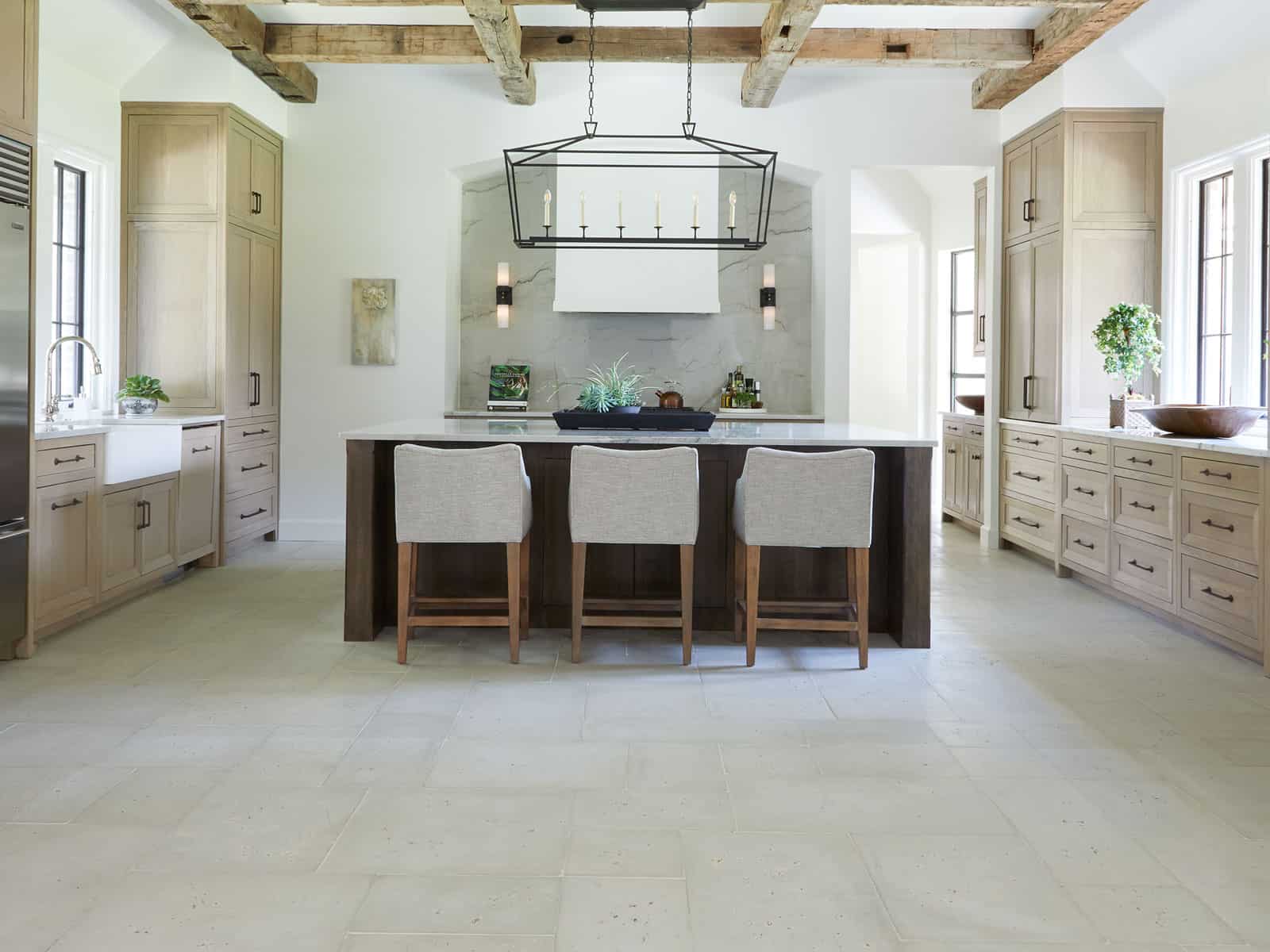This horizontal rectangular photograph captures the interior of an expansive, vintage English farmhouse-style kitchen. Dominating the room is a large central island table with a lacquered or marble top, offering ample space that rivals the size of some apartments. Surrounding this are meticulously crafted light-colored wood grain cabinets and drawers, creating a seamless, uniform look throughout the kitchen. On the left side, a prominent cabinet stands, accompanied by smaller shelves, while the right side boasts more cabinetry, a large bowl atop one, and two windows that illuminate the space.

The kitchen also features a deep, farmhouse-style sink with a gleaming, modern faucet located on the right. Above, sturdy wooden beams—reminiscent of an old barn—criss-cross the ceiling, providing a rustic charm. There are four beams running one way and two beams intersecting them. Hanging from these beams is a metal tray light fixture designed with candlestick lights, adding to the vintage aesthetic.

A marble backsplash highlights the cooktop area, nestled within a grand arch alcove that further enhances the room's farmhouse appeal. The light tiling and whitewashed walls brighten the space, creating a welcoming atmosphere despite the absence of inhabitants. Overall, the photo encapsulates a beautifully detailed and spacious vintage kitchen, marrying modern functionality with rustic design.